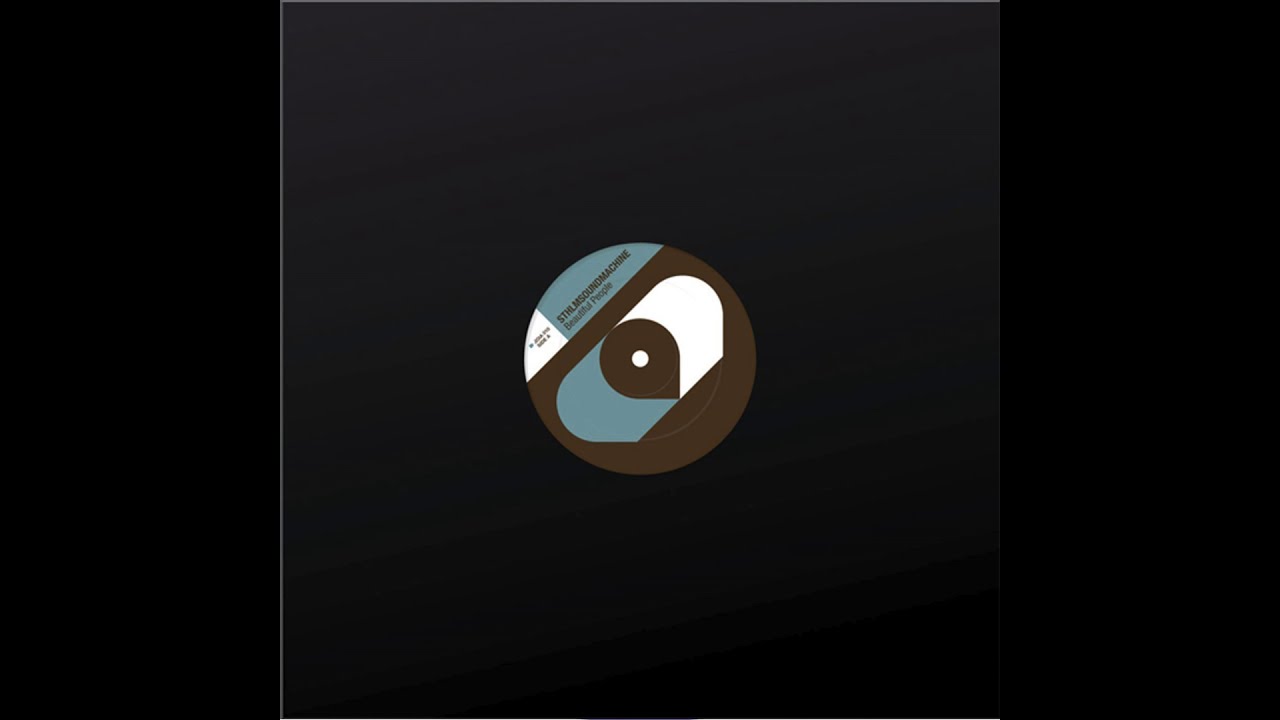The image is a likely album cover presented as a square with a solid, very dark gray background. Central to the design is a circular disk reminiscent of a record label, featuring intricate gray and white patterns. The text on the disk, written entirely in capital letters, ends with the word "MACHINE" and includes the phrase "BEAUTIFUL PEOPLE." However, the text is largely illegible due to its small size. The overall color palette includes three shades of black, as well as touches of white and blue. The central focus is the disk, seamlessly integrated into the middle of the square background, creating a minimalist yet striking design meant to evoke the aesthetic of a classic record album.